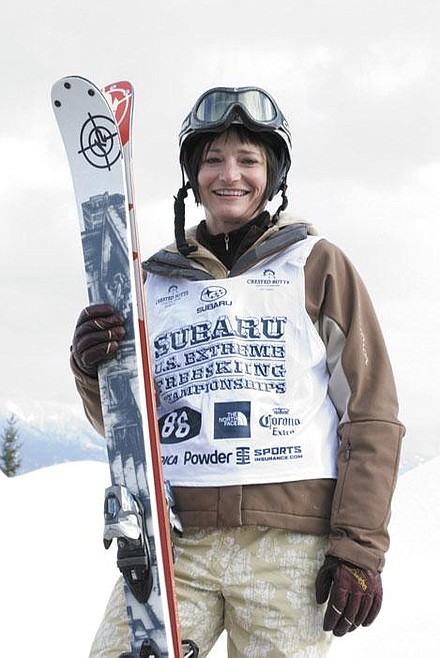This photograph features a female skier standing on a snowy mountain, gazing directly at the camera with a smile. She is clad in ski attire, including a brown zip-up snow jacket layered under a white vest bearing multiple sponsorship logos such as Subaru U.S. Extreme Free Skiing Championships, her contestant number 86, The North Face, Corona Extra, and what appears to be sportsinsurance.com. Her gear also includes brown gloves and tan ski pants with a white pattern. She’s holding a pair of skis in her right hand – one notably red with a gray pattern and the other white with a blue pattern. Her ski goggles, a reflective silver, rest above her dark brown bangs. The backdrop showcases an expansive, overcast gray sky, snowy slopes, and a distant pine tree to the left, accentuating the wintry setting of the ski championship.